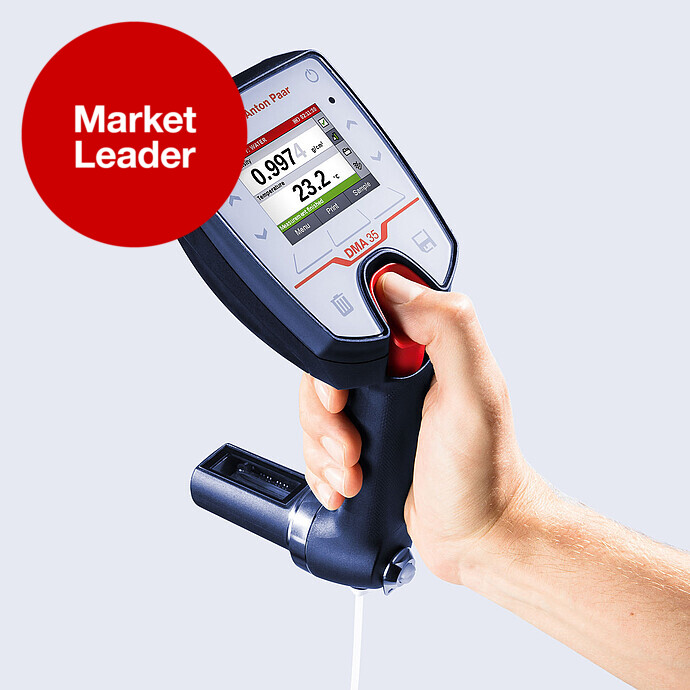The image depicts a unique measuring device resembling a combination of a joystick and a rectangular panel with an LCD screen. The device, held by a disembodied arm extending from the bottom right corner of the frame, is made of navy blue material and features a prominent red button at the top. The screen displays a temperature reading of 23.2 Celsius, with additional gauges and buttons flanking the display on the left and right sides. A large, bold red circle in the upper left-hand corner of the image contains the words "market leader" in white lettering. The background is simple and gray, possibly indicating a studio setup or a digitally altered image. This instrument, potentially labeled as an Anton Parr device with a model number DMA35, could be used for health-related measurements, possibly including pulse or oxygen levels.